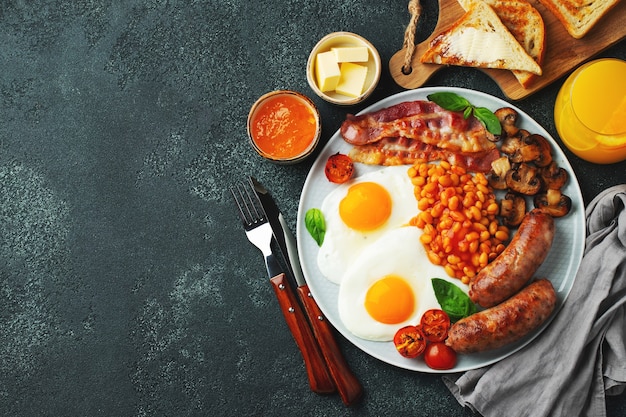The image is a top-down view of a beautifully arranged traditional British fry-up breakfast set against a charcoal grey textured surface, perhaps a countertop. Dominating the right side of the landscape-oriented photograph is a circular plate featuring a light blue hexagonal pattern. The plate is laden with two sunny side up eggs, two sausages, baked beans, sautéed mushrooms, two rashers of bacon, and a few cherry tomatoes, all garnished with basil leaves. Accompanying the plate are a glass of orange juice to the right and a wooden breadboard topped with buttered toast at the top edge. A small ramekin with three pats of butter and another with a red sauce sit just above the plate. To the bottom right, there is a neatly folded grayish-blue napkin. On both sides of the plate lies a stainless steel knife and fork, adorned with red wooden handles, ready for use.